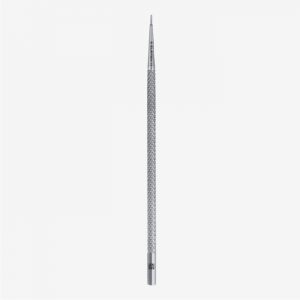The image depicts a slender, metallic object that might be a pen or stylus, standing upright against a very light, possibly blue, background. The pen-like instrument spans about 8 inches in height, characterized by a grooved grip in the middle and a pointed tip, suggesting possible use as either a writing tool or a pointer for presentations. The object’s body is primarily silvery gray, with a darker hue towards the top, culminating in a sharp point. The base appears to have a clearer silver tone with a small white dot or hole. The sleek, shiny design and grooved texture create an aesthetic yet functional appearance, though the image is small and lacks textual details.